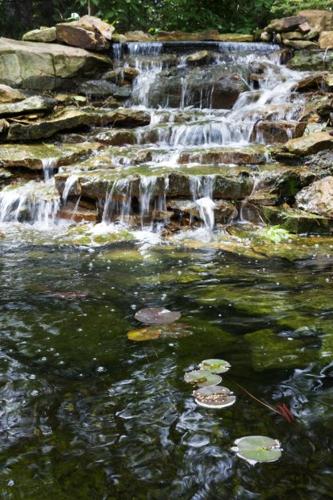This vertical photograph captures a small, cascading waterfall on a bright, sunny day. The waterfall, situated at the top of the image, flows down a series of about 7-10 rocky steps, creating a white rapid effect as the water crashes down. These stacked, brown rocks form a natural staircase that leads into a pond partially visible in the frame. The pond's surface, dotted with lily pads, reveals a greenish hue, likely due to algae on the submerged rocks. In the background, hints of trees and greenery frame this tranquil scene, adding to the overall peaceful and serene atmosphere of the image. The water's color transitions from darkish green in the deeper areas to a lighter shade near the waterfall, enhancing the sense of depth and natural beauty.